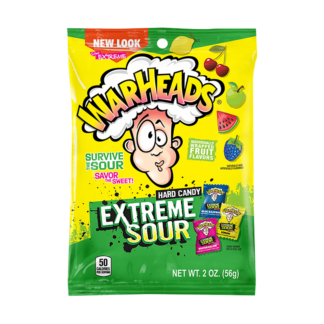The image depicts a close-up of a vibrant package of Warheads Extreme Sour Hard Candy, positioned vertically against a white background, resembling a stock photo. Dominated by a yellow and green color scheme, the top portion of the bag is primarily yellow, transitioning to green at the bottom third. A green tab is visible at the top, along with a prominent red flag proclaiming "New Look."

Centrally placed on the packaging is the iconic Warheads logo within a cloud, featuring a comical, cartoon-like face with exaggerated eyes and pursed lips, giving a visual representation of sour intensity as if his head is about to explode. Surrounding the logo are illustrations of various fruits including a cherry, green apple, watermelon slice, purple grapes, yellow lemon, and blueberries, symbolizing the candy’s assorted flavors.

The bag elaborates the challenge and experience of the candy with phrases like "Survive the Sour," "Savor the Sweet," and reiterates "Hard Candy, Extreme Sour" in the green section at the bottom. Three smaller images depict individual candies in blue, yellow, and pink wrappers with needle-point edges, noting their easy-to-tear design. Additionally, the bag indicates it contains 50 calories and has a net weight of 2 ounces.